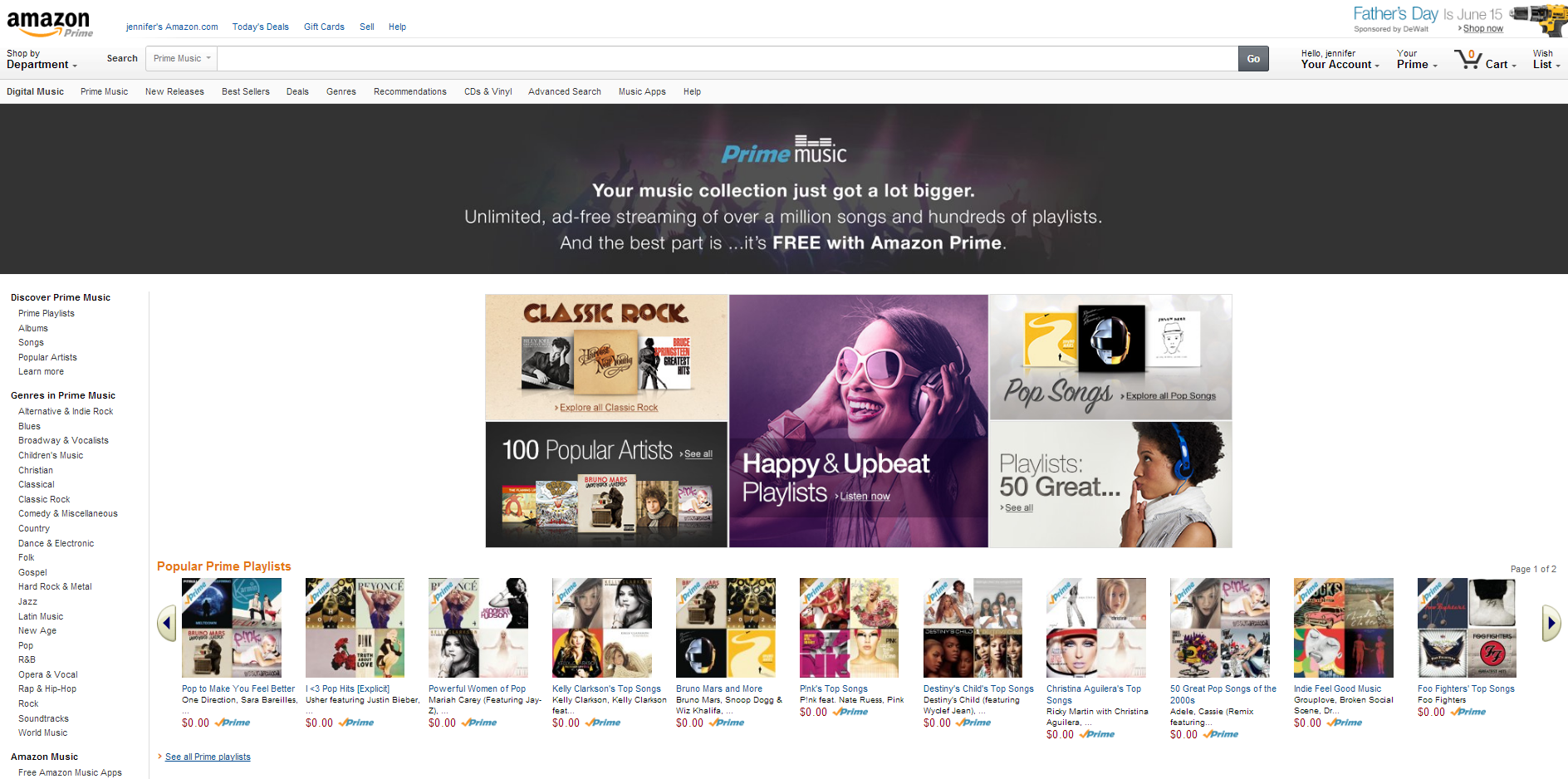The screenshot captures a desktop view of the Amazon website in Prime mode, specifically highlighting the Prime Music feature. At the top of the screen, there’s a prominent banner stating, "Your music collection just got a lot bigger," accompanied by an advertisement for Prime Music. Below the banner, various music categories and playlists are displayed, each represented by different-sized icons. The categories include "Classic Rock," "100 Popular Artists," "Happy and Upbeat Playlists," "Pop Songs Playlists," and "50 Great."

Further down, there is a long row labeled "Popular Prime Playlists" featuring curated playlists such as "Pop to Make You Feel Better," "I Love Pop Hits," "Powerful Women of Pop," "Kelly Clarkson's Top Songs," "Bruno Mars and More," "Pink's Top Songs," "Destiny's Child's Top Songs," "Christina Aguilera's Top Songs," "50 Great Pop Songs of the 2000s," "Indie Feel-Good Music," and "Foo Fighters Top Songs." To the right of these playlists, an arrow indicates the option to see more, signifying that this is page one of two.

On the left side of the screen, a sidebar lists music categories available on Prime Music, such as "Alternative and Indie Rock," "Blues," "Broadway and Vocalists," "Children's Music," and several others. In the upper right-hand corner, there’s a reminder that "Father's Day is June 15th" accompanied by an image of a drill, adjacent to the account name, "Jennifer."